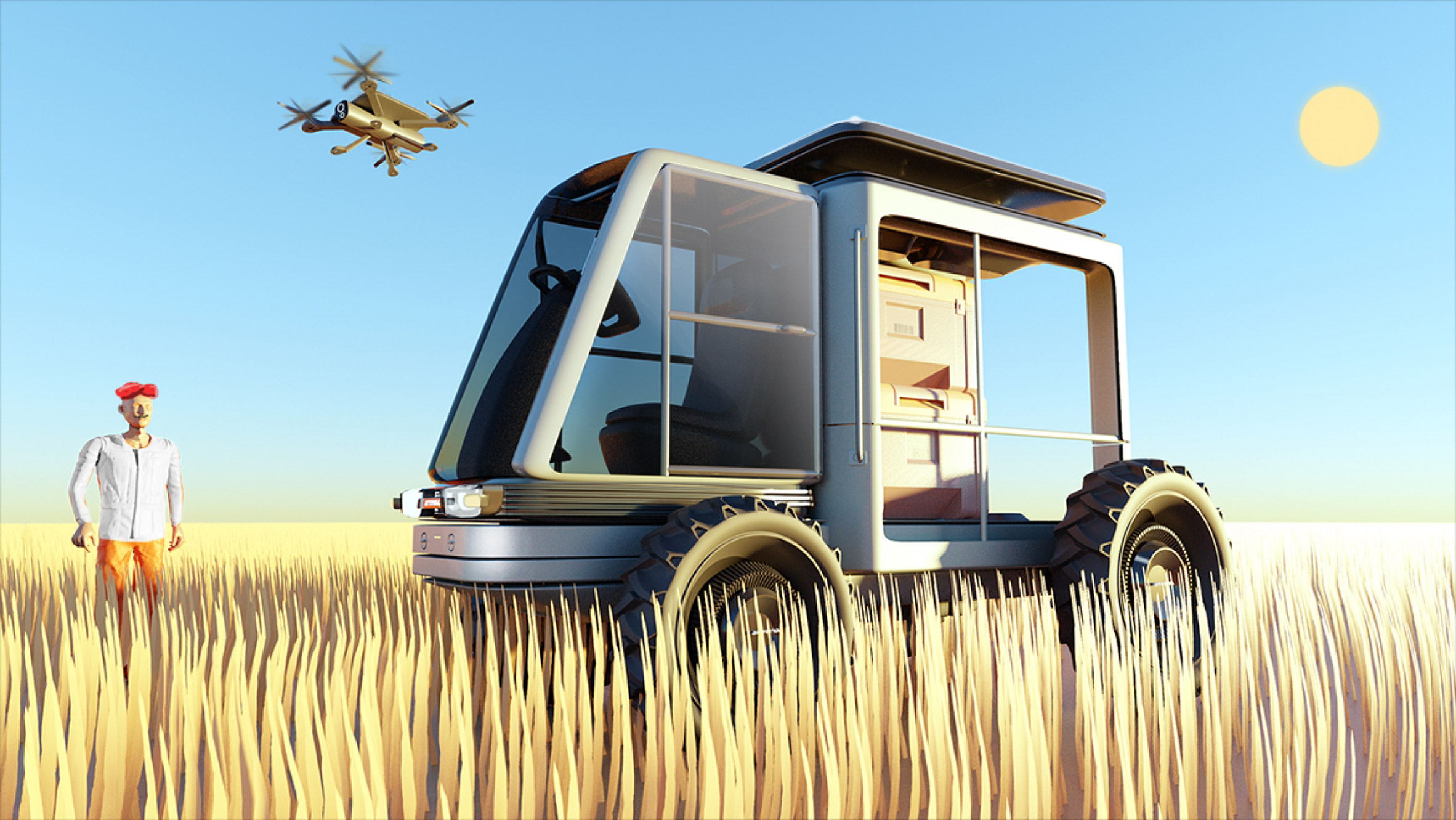The image is a digitally created outdoor scene set in a vast wheat field, characterized by long strands of yellow and brown grass mixed with patches of white. Dominating the center is a man dressed in orange pants, a white button-down shirt, and a red cap. He has a mustache and is visible from about mid-thigh up. To his right stands a futuristic-looking vehicle with an enclosed front area, large glass pane, and four wheels. The back end of this vehicle is squared and open, with what appears to be a solar panel on top. Overhead, a square drone with propellers on each of the four corners flies in a sky painted light blue, underlining a small, round yellow sun positioned in the upper right-hand corner. The scene captures the harmonious blend of agricultural life and advanced technology under a bright, sunny day.